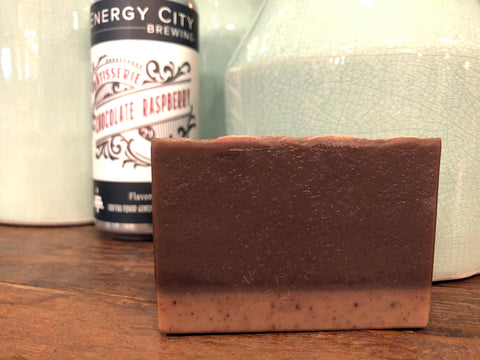This detailed photograph captures a unique arrangement of items on a textured, brown wooden surface. Centrally featured is a distinctive rectangular soap, narrow in thickness, presented in a dual-color scheme. The soap showcases a larger, darker brown or reddish-brown upper section, transitioning into a smaller, pale orange or beige base. Behind this intriguing soap lies a bottle of beer from Energy City Brewing, known for its Chocolate Raspberry flavor. The bottle is primarily dark blue and white, with its brand and flavor text elegantly written in red and white. Accompanying these items, the background reveals several white porcelain jars, adding a touch of sophistication to the scene. The whole setting, blending personal hygiene products and an artisanal brew, creates a curious and visually appealing still life.